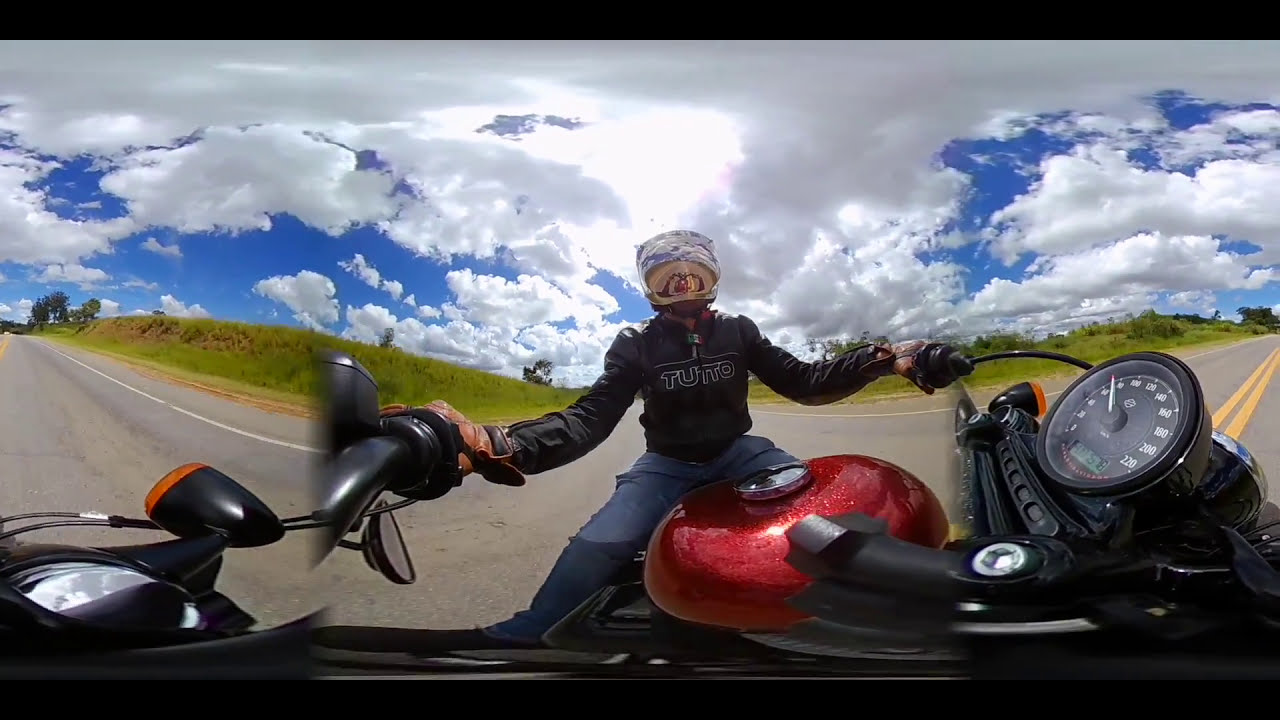A detailed selfie image captures a motorcyclist riding a metallic red motorcycle along a light gray asphalt road with clear yellow center lines and solid white edge lines. The motorcyclist is clad in a distinct outfit, featuring gray pants, a padded black leather jacket with white text reading "Toro" or "TUTTO" on the front, and brown leather gloves firmly gripping the black handlebars. Their head is protected by a striking helmet exhibiting white, blue, and possibly silver or gold hues with a reflective visor obscuring their face. Additionally, the motorcycle's dashboard is visible, showing black gauges with white numbers, possibly indicating a speed range of 60 to 80 kilometers per hour. The scene is set against a vibrant, expansive green field that slopes upward towards a hill, with a patch of blue sky overhead filled with puffy white and gray clouds, suggesting a sunny day with some cloud cover. No other vehicles or people are present in the image, highlighting the lone rider in this picturesque and dynamic moment.